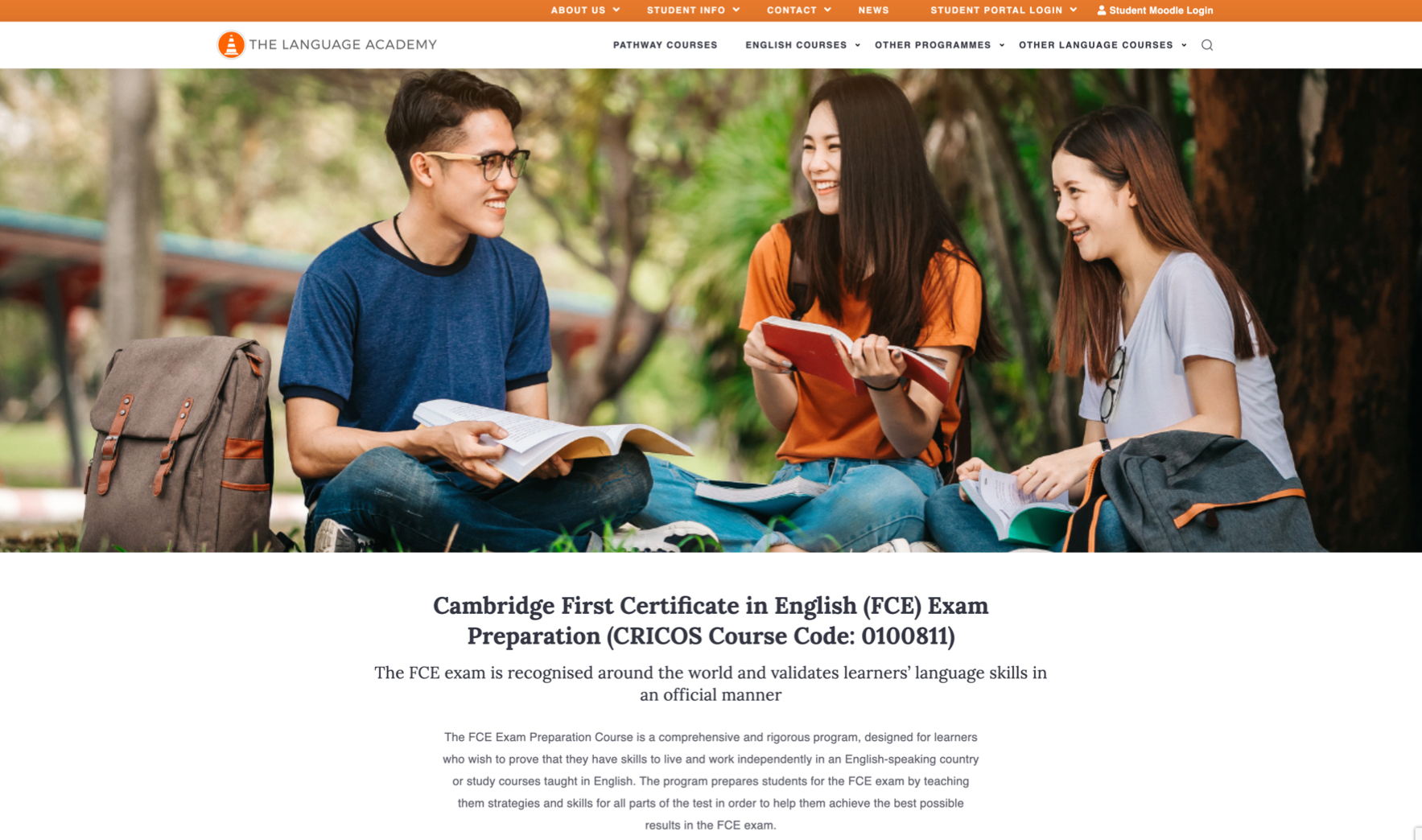The webpage featured in the image belongs to an institution named the "Language Academy," potentially associated with Cambridge. The top navigation bar has an orange background and includes links such as "About Us," "Student Info," "Contact," "News," and "Student Portal Login." As you scroll down, additional links are displayed against a white background, directing users to pages on "Pathway Courses," "English Courses," "Other Programs," and "Other Language Courses," suggesting that this program is catered specifically for international students aiming to learn English.

Centrally featured on the page is a stock photo depicting three Asian students—a male and two females—socializing in an open outdoor area. They are all engaged and cheerful with books open in front of them. Below this image, there's a section dedicated to the "Cambridge First Certificate in English" (FCE) exam, detailing how this globally recognized exam officially validates the language skills of learners. The bottom of the page contains a variety of legal information. The overall design aesthetic of the webpage includes a white main background and black text.